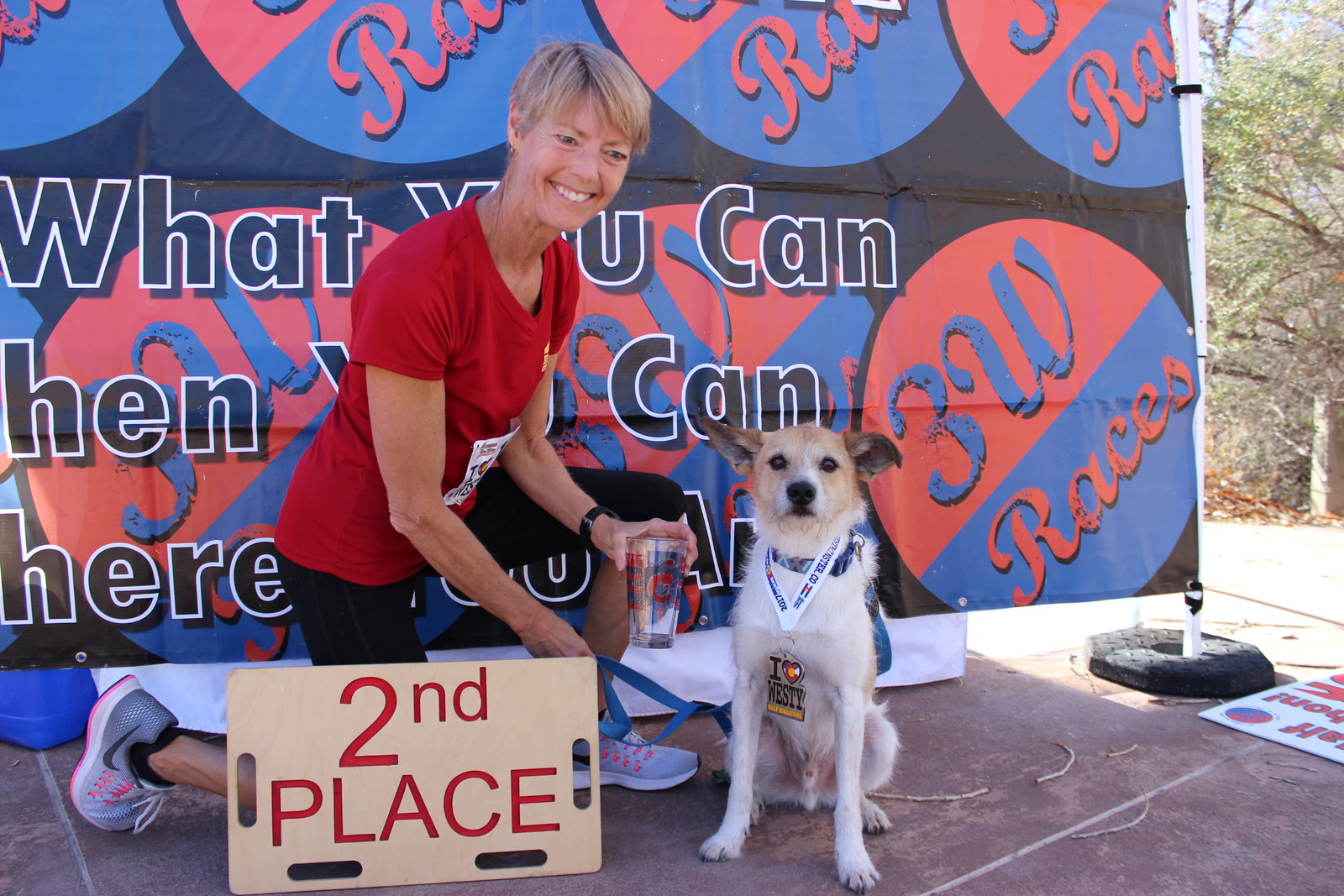In the outdoor photo, a woman in her 50s or early 60s with short blonde hair, is kneeling on one knee, smiling while looking down at the ground. She is wearing a red T-shirt, black capri pants, and Nike sneakers. She holds a clear plastic cup in her left hand and a blue lead in her right, which is attached to a male dog sitting beside her. The dog, who is looking directly at the camera, has a brown head, black nose, white and brown fur, and a medal around his neck that reads "I Heart Westy." In front of the woman, there is a square wooden sign that reads "Second Place" in red letters. Behind her, a larger sign has the slogans "What You Can, When You Can, Where You Can" and "3W Races" amidst red and blue circles. The backdrop and her attire suggest she might have participated in a running event.